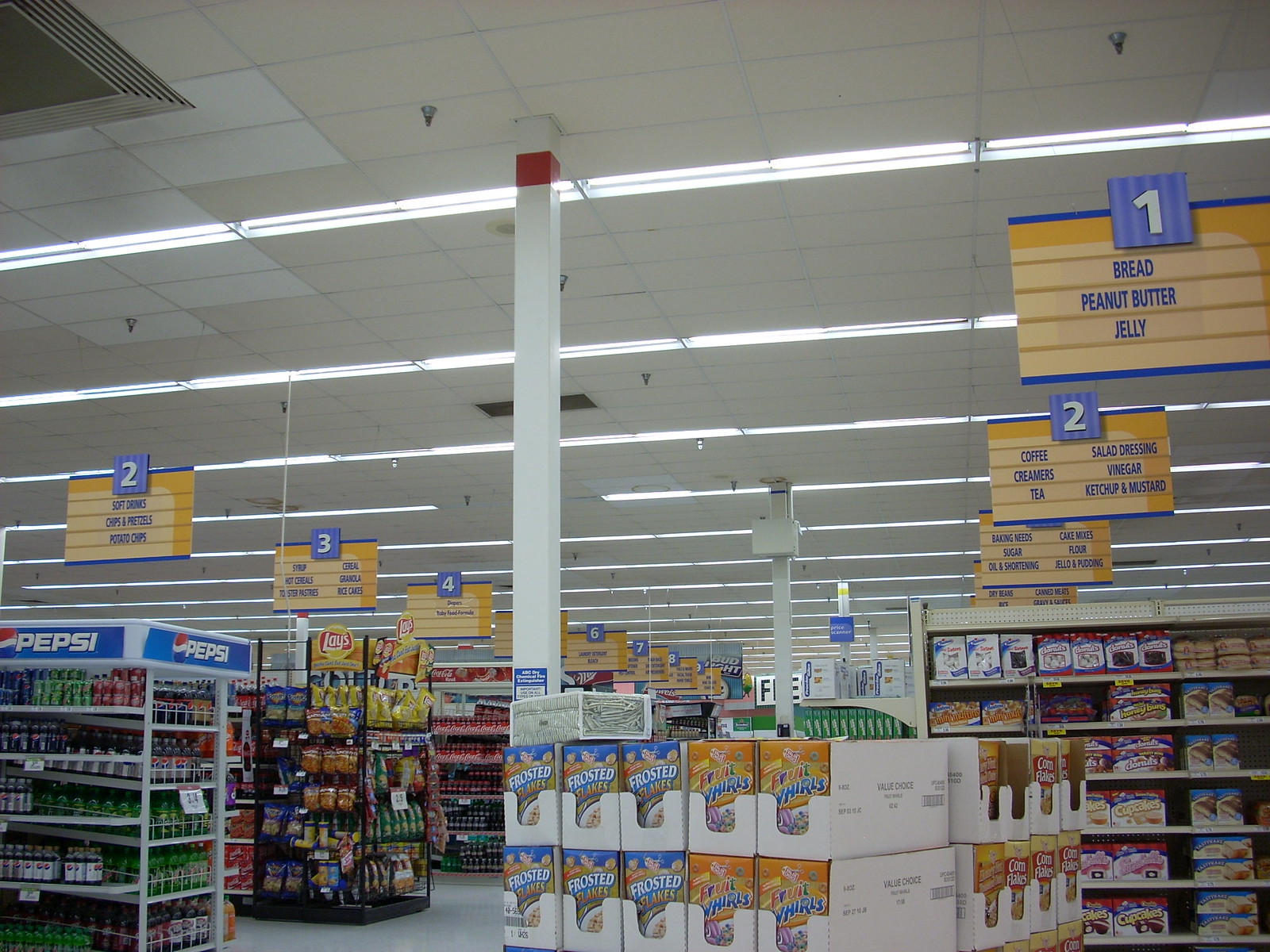In the image, there is a well-organized grocery store aisle. Centrally displayed are neatly stacked cereal boxes, creating a vibrant focal point. Flanking the cereal section are various aisles, each demarcated by hanging yellow signs indicating their contents. These signs are topped with blue squares featuring aisle numbers in prominent blue text. Aisle one is dedicated to bread, peanut butter, and jelly, while aisle two contains coffee, salad dressing, vinegar, ketchup, and mustard. The left aisle also includes coffee creamers and tea. The store’s interior design includes a white tiled floor and a similarly white ceiling adorned with grid-like wooden panels. The ceiling also features several strobe lights and a few sprinkler systems, ensuring both illumination and safety within the store.